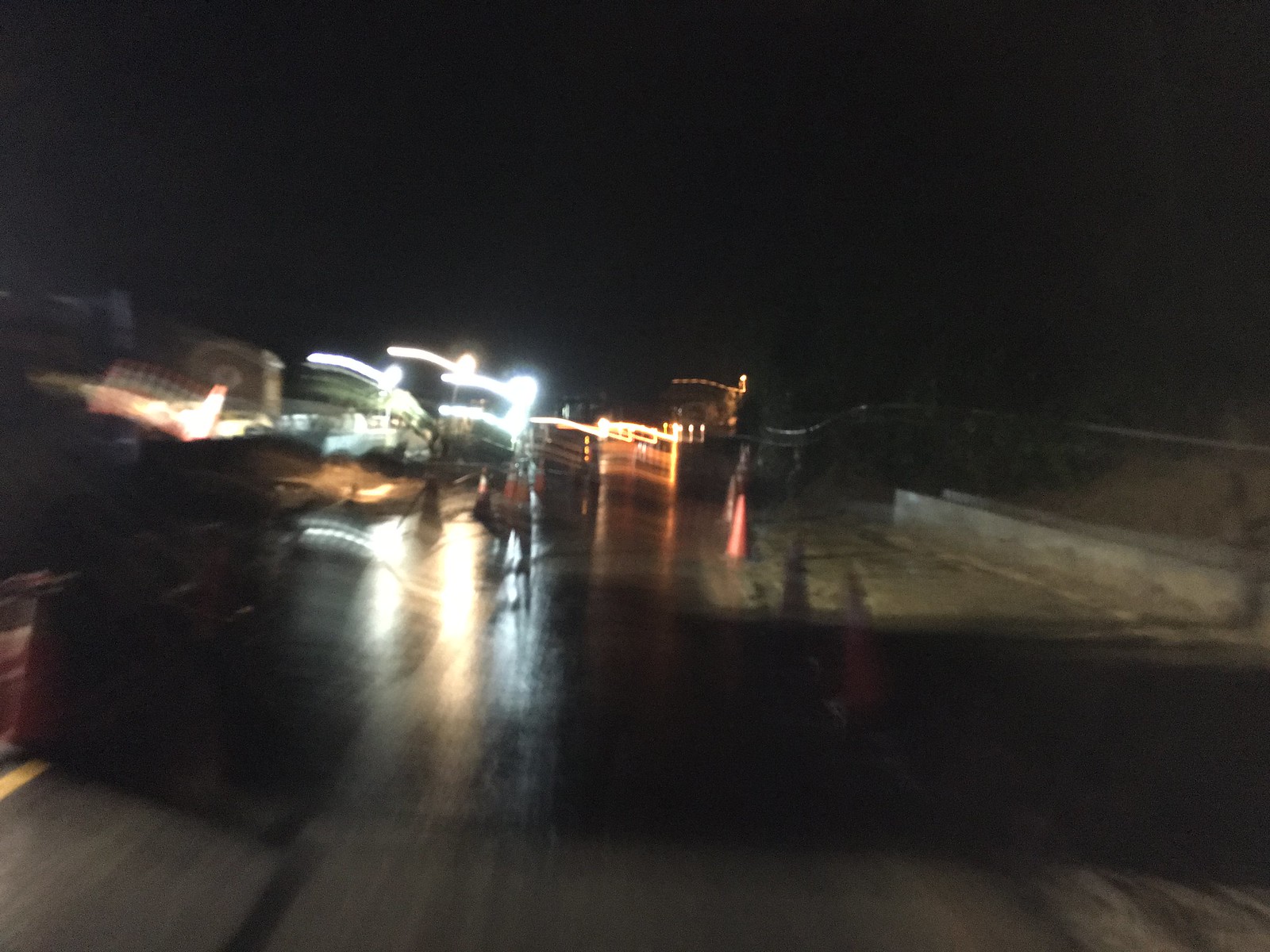This image is a color, landscape-format photograph taken outdoors at night. The photograph is blurry due to motion and a slow shutter speed, which creates a sense of movement and makes specific details difficult to discern. The background is dominated by a black night sky, indicating the time of day. The foreground features a largely flat, concrete surface, possibly a road or construction site, which appears to be wet as evidenced by the numerous reflections of various distant lights on its surface. 

Several orange construction cones are scattered across the scene, suggesting a work zone on a public roadway. Bright lights from construction equipment and vehicles are visible, though they are blurred and create streaks of light across the image. These vehicles and their lights, including what might be white headlights and red taillights, hint at activity but are not clearly identifiable. There may also be a figure standing near the center of the image, potentially a policeman or construction worker, adding a human element to the nighttime work scene. The right side of the photo shows cement jersey barriers, reinforcing the idea of a construction or maintenance area. Despite the low resolution and motion blur, the image conveys the chaos and activity of a nighttime road work zone.